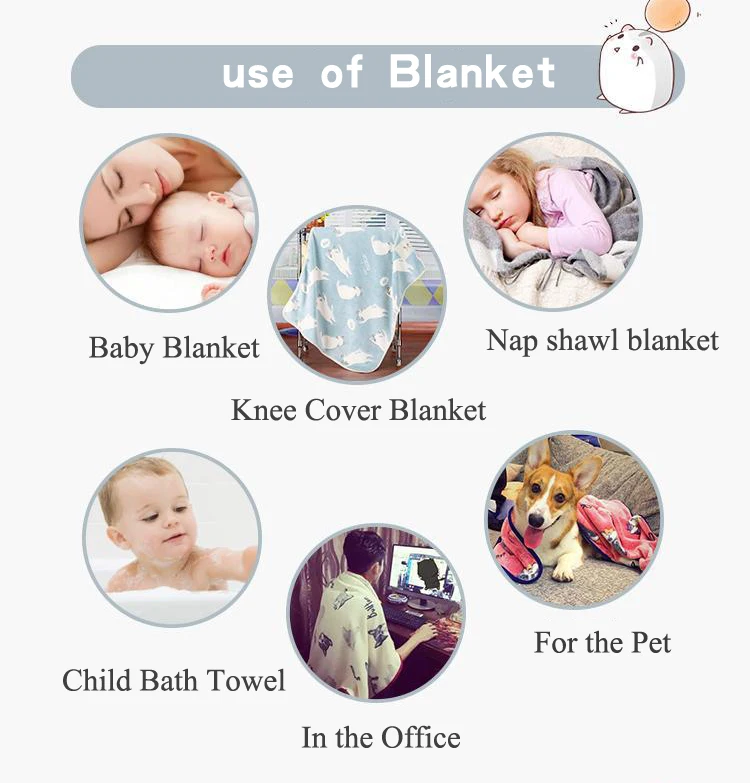This digitally created graphic, titled "Use of Blanket" in white letters across a gray banner at the top, features a whimsical cartoon hamster with a white stomach, holding a peach-orange balloon in the upper right corner. The graphic is divided into two rows of three centered circles, each depicting different uses for a blanket. From left to right on the top row: a mother and baby sleeping, labeled "Baby Blanket"; a blue blanket with white graphics, labeled "Knee Cover Blanket"; and a young girl in a purple shirt sleeping, labeled "Nap Shawl Blanket". On the bottom row, from left to right: a child in a bathtub, labeled "Child Bath Towel"; a person sitting at a computer with a blanket around their shoulders, labeled "In the Office"; and a brown and white dog on a couch covered with a pink blanket, labeled "For the Pet". The background is predominantly white, adding to the clean, organized presentation of the colorful images, which include shades of gray, white, light blue, pink, tan, light purple, peach, and black.